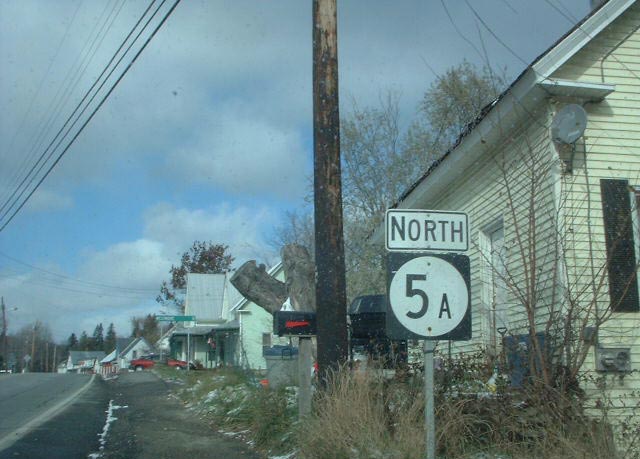This color photograph captures a slightly dreary scene of a small town. Dominating the image are a series of lackluster homes and possibly some small businesses, characterized by their tired vinyl siding and somewhat overgrown yards. A bit of an unkempt, two-lane road runs parallel to these structures, identified as Highway North 5A by a prominent street sign. In the foreground, a utility pole stands with its wires stretching across the frame. The general landscaping is scruffy and undeveloped, with the homes positioned close to the road. The sky overhead is mostly cloudy, featuring some stormy-looking clouds that add to the overall gloomy atmosphere.